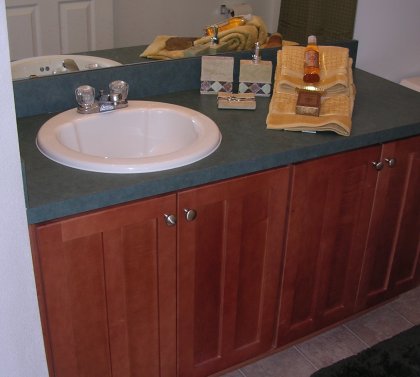The image captures a detailed view of a bathroom. At the center is a white sink with two clear handles situated on top of it, along with a silver metal faucet. The countertop has a dark bluish hue, complementing the metallic fixtures. On the countertop, there is a gray soap dispenser adorned with diamond patterns, accompanied by a small tray holding a bar of soap. To the right of the sink, a yellowish towel is visible, topped with an orange bottle of soap and a smaller, indistinguishable box.

The mirror above the sink reflects several details, including a white door and some drapes. Below the sink are brown wooden cabinets, and the bathroom floor is made of stone. In the bottom right corner of the image, a dark-colored rug can be seen, adding a final touch to the room’s decor.